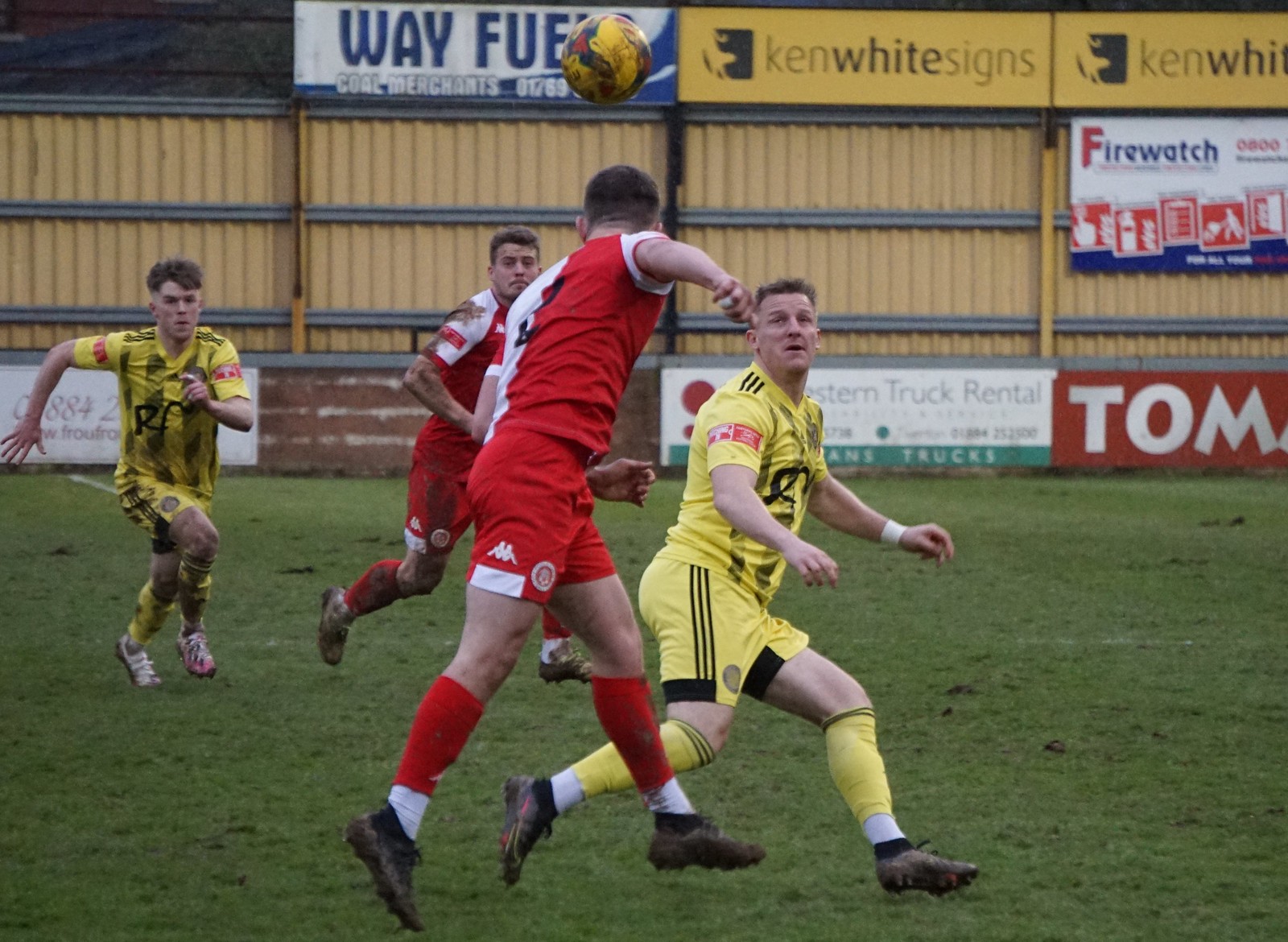The photograph captures a lively soccer match taking place in what appears to be an older stadium, devoid of typical spectator stands. The background is marked by a distinctive yellow tin fence, which, along with some advertisements such as the white and blue "Wave Fuel" and the yellow and black "Ken White Signs," lends a unique character to the setting. The field is green but noticeably worn, with patches of dirt visible. Four players are prominently featured: a player in a red and white uniform is actively heading a yellow and blue ball, facing away from the camera. Directly behind him, another player in red and white faces the camera. To the right, a player in a yellow and black uniform stands out, while another yellow-and-black-clad player is seen running towards the camera on the far left. The players in yellow and black also have detailed uniforms with black piping and designs, complemented by red flags or advertisements on their shoulders.